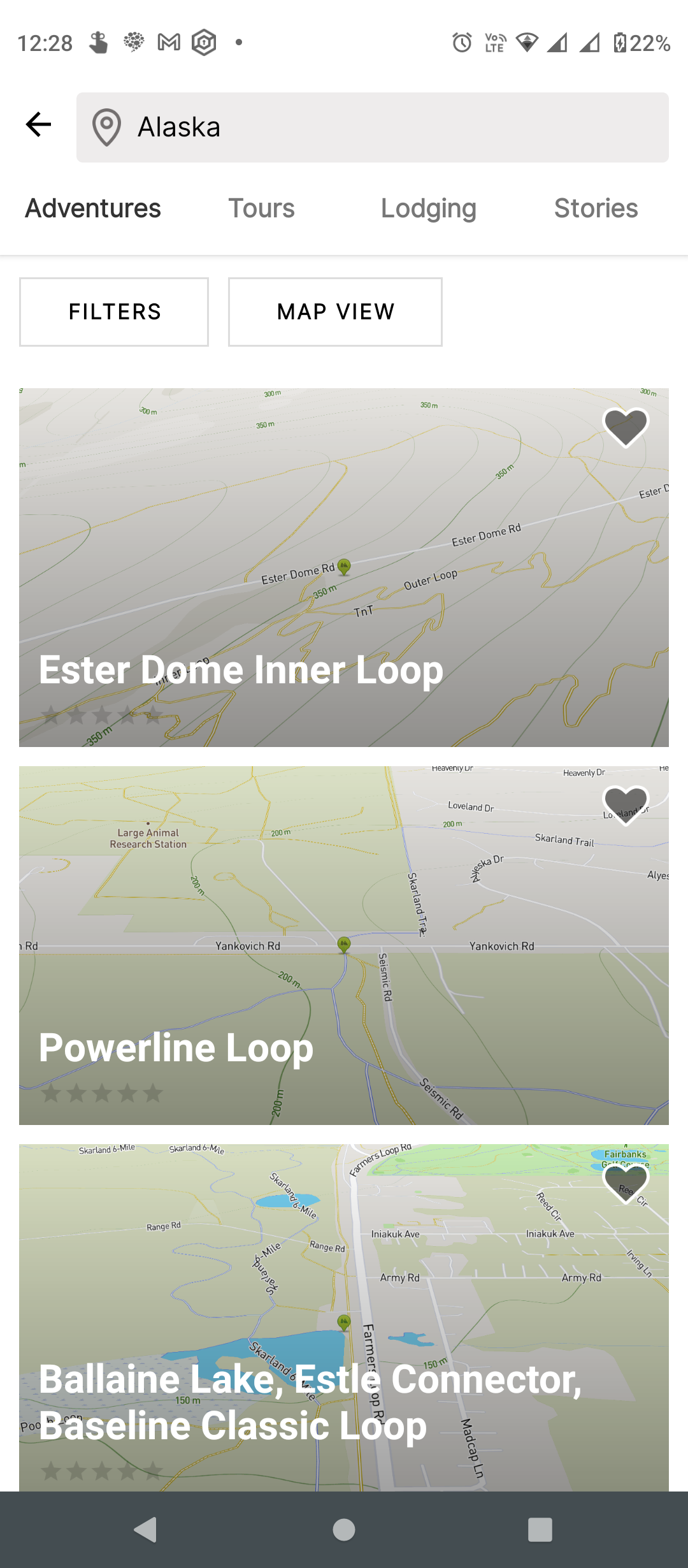**Detailed Caption:**

This image is a screenshot from a mobile phone, captured at 12:28 PM. The status bar indicates various icons including a handprint or a pointer finger icon, a speech bubble icon, an "M" icon, a sideways Pokéball-like icon, and a hexagonal icon alongside a dot. The alarm clock is active, and "V-O-L-T-E" is displayed, suggesting voice over LTE service. The phone shows decent Wi-Fi and service connectivity, with a battery level of 22%. The current location or search query appears to be set to Alaska. The search bar is accompanied by a location tag. 

Below the search bar, "Adventures" is prominently bolded, with "tours," "lodging," and "stories" in slightly less bold font. Options for "filter" and "map view" are highlighted within light gray rectangles, indicating interactive elements. The phone is in daytime mode, featuring a white background with lighter colored fonts. 

The displayed content includes three different maps. The first map highlights the Easterdome Interloop, with Estherdome Road being the main road featured. Other highlighted routes include the Power Line Loop and Yankovitch Road near the Large Animal Research area. The second map shows Belain Lake, Estale Connector, and Baseline Classic Loop with Farmer's Loop Road as the main road.

Each map fragment presents detailed routes and landmarks, offering an organized view of the adventurous terrains within Alaska.